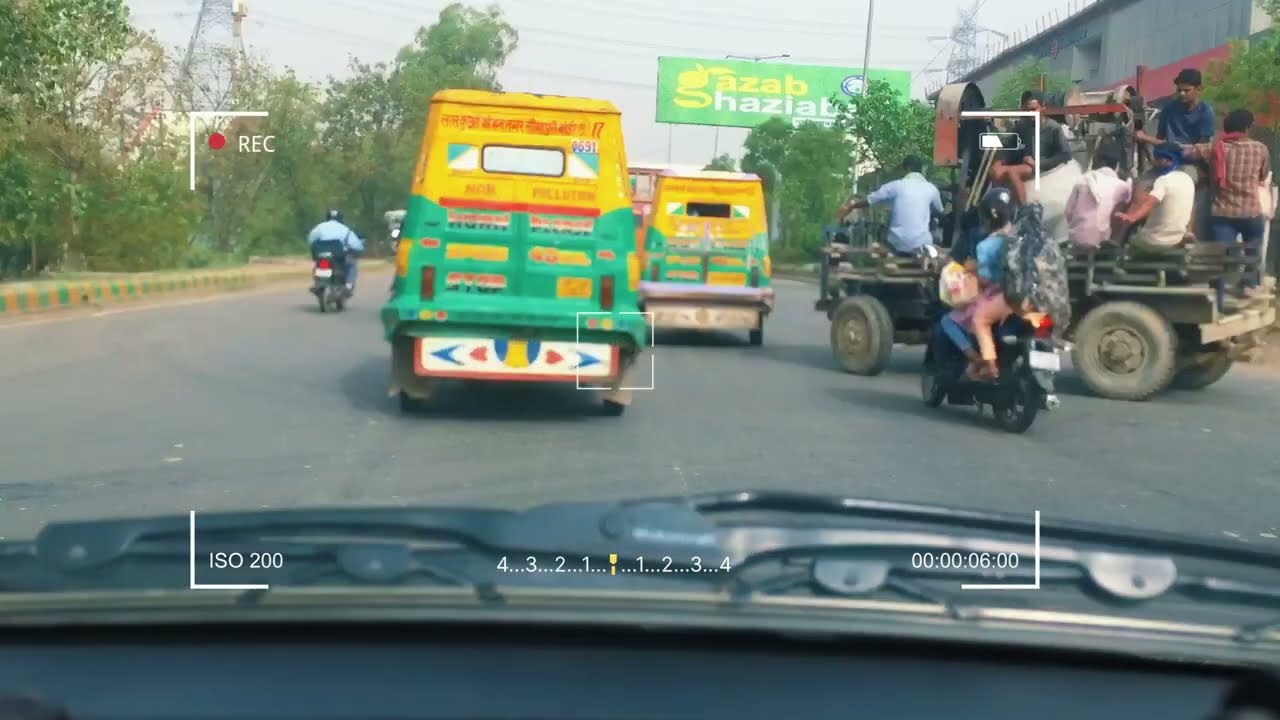The image, taken from a dashboard cam inside a vehicle, shows a wide street scene during the daytime with several distinct elements. The camera captures part of the vehicle's windshield, dashboard, and the hood, as well as some dashboard cam interface details like recording information and a timer. Directly ahead on the road are two identical vans, vividly painted with green on the bottom and yellow on the top, adorned with various writings and symbols. In the middle of the image, between the two vans, a colorful flag with distinct blue and red elements can be seen on the back of one of the vans. To the right of these vans is a small, black motorcycle carrying two passengers— a likely female driver and a small child seated behind her, both wearing helmets. Nearby, a packed open-bed Jeep loaded with around eight to ten people is visible, while on the far left of the street, another motorcycle, ridden by a man in a blue shirt, travels alongside. Flanking the scene, trees line the left side of the road and there's a tall, dark, blue stone building on the right.